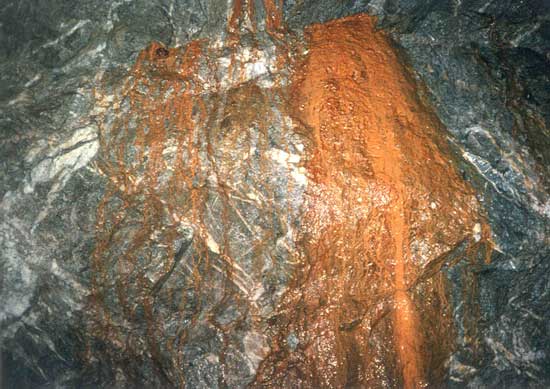In this image, a highly textured rock surface, resembling granite with a shiny black, white, and occasionally pinkish hue, is prominently displayed. The rock's intricate pattern is characterized by numerous thin white lines crisscrossing the dark background. Overlapping this striking base, brown streaks, appearing similar to rust or an orangey-brown clay, cascade down the surface. These streaks are more densely concentrated on the right side, obscuring the underlying rock almost entirely in that area. In the middle and left sections, the brown streaks are thinner and more sporadic, allowing the distinct pattern of the black and white rock to remain visible. The combination of the shiny textured rock and the contrasting sediment creates a visually complex and detailed image.